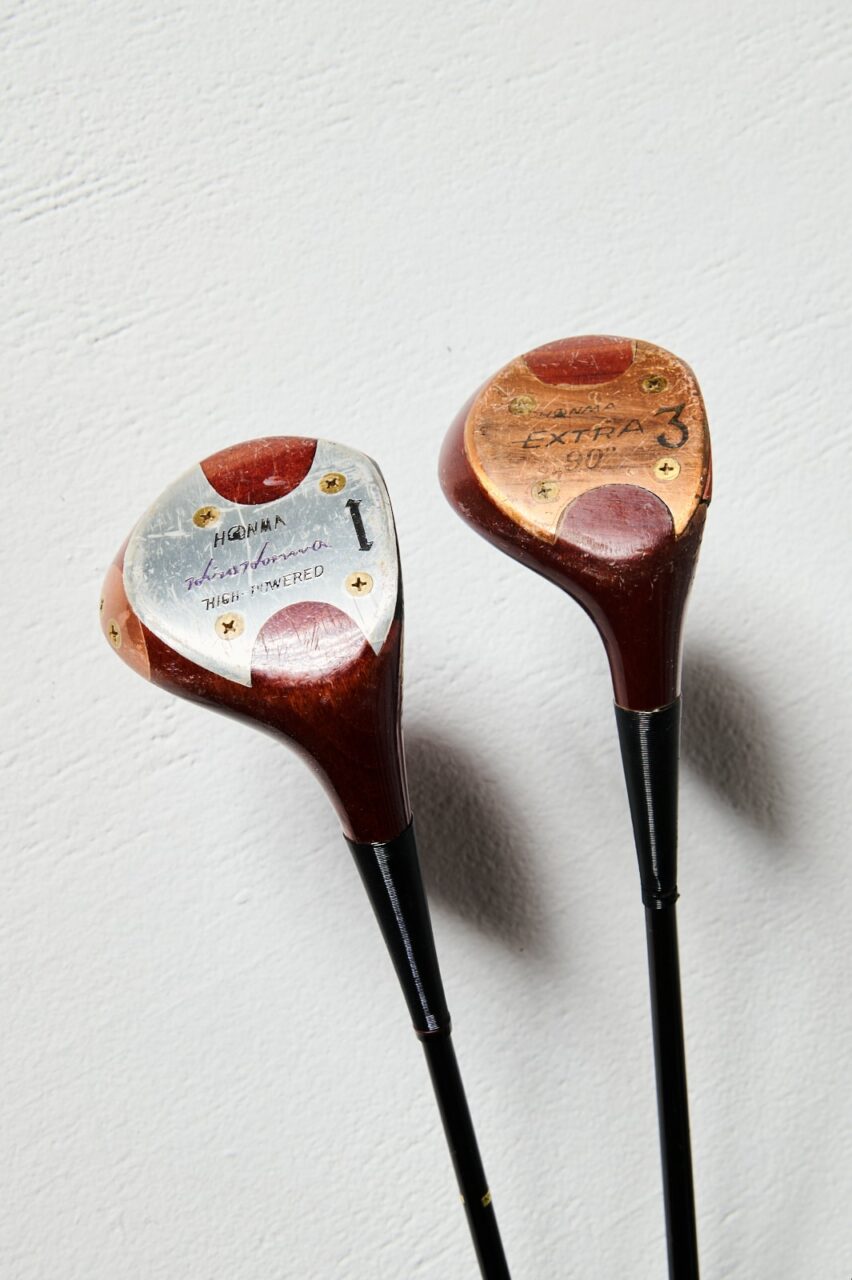This indoor close-up photograph showcases the bases of two vintage golf clubs leaning against a white wall. The club on the left has a black shaft leading up to a wooden base with a silver metal plate, secured by four bronze screws. This club features inscriptions including "HG one," a signature-like marking, and the phrase "high powered." The club on the right also has a black shaft and a wooden base but is fitted with a bronze metal piece attached similarly with four bronze screws. The inscription "extra 390" and a number "3" are visible, though some text remains illegible. Both clubs, appearing worn and old-fashioned, highlight the craftsmanship and materials of earlier golfing equipment.